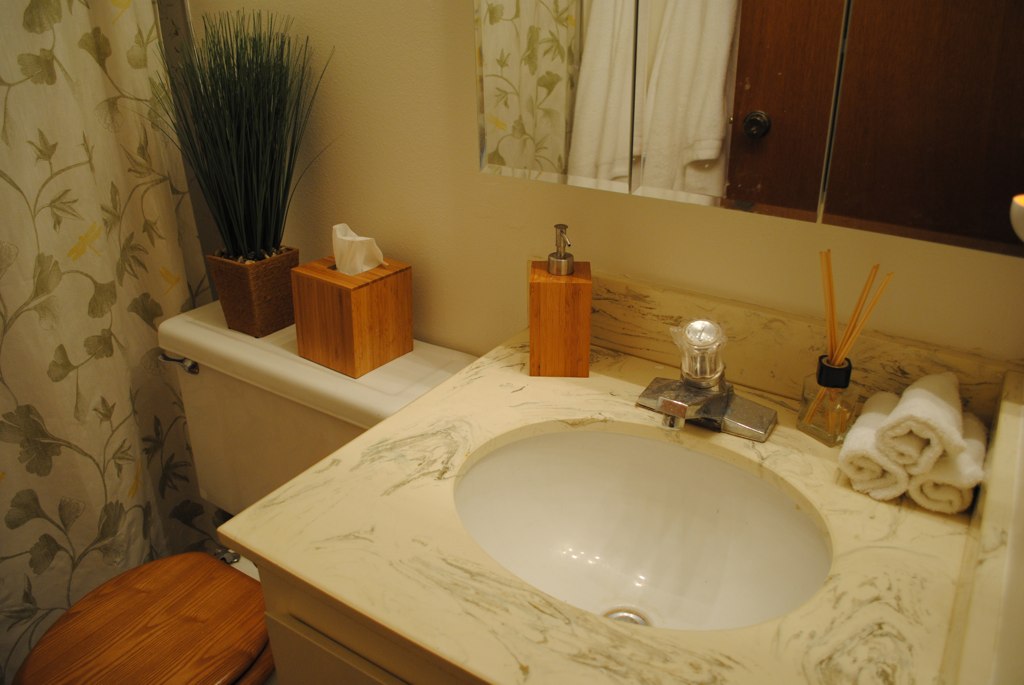This photograph captures a well-organized washroom with a soothing, neutral aesthetic. The creamy beige walls set a warm backdrop. In the top-left corner of the image, a mirror reflects a brown door, complete with a matching brown handle, and something white hanging from it. 

In the bottom right-hand corner, a pristine white sink with silver fixtures sits upon a cream-colored countertop adorned with subtle swirls. Three neatly rolled towels are situated in the countertop’s corner, enhancing the space's tidy appearance. A sleek, silver faucet features a modern white handle. Continuing the countertop’s decor, a glass jar filled with incense is positioned next to a wooden soap dispenser that sports a stylish silver top.

To the left of the sink, a white toilet with a brown wooden seat adds to the natural decor theme. Atop the toilet's tank, there is a wooden box containing a Kleenex box, alongside a potted plant in a brown pot, bringing a touch of greenery to the setting. Towards the far left of the photograph, a shower curtain adorned with green leaf patterns extends the room's cohesive color scheme.